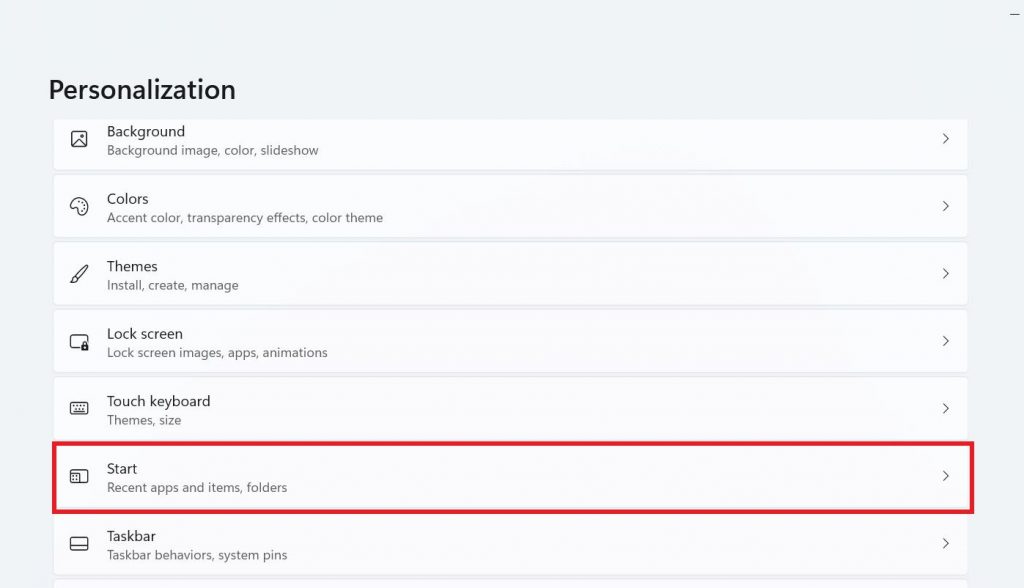The image depicts a Windows personalization menu, characterized by a light grey background and predominantly white interface with black text. At the top left, "Personalization" is prominently displayed in large font. Below this heading, there is a series of white rectangles each accompanied by thin greyish background bars and small forward arrows on the right side. 

Each rectangle includes an icon followed by text. The first rectangle, labelled "Background," encompasses options such as background image, color, and slideshow settings. The second rectangle features a painter's palette icon and the word "Colors," offering customization for accent colors, transparency effects, and color themes.

The third rectangle, marked by a paintbrush icon, is labeled "Themes," and provides options to install, create, and manage themes. Following this, "Lock screen" manages settings like lock screen image, apps, animations, and touch keyboard themes.

One section, partly obscured, seems to address the date settings, but it remains unclear due to its small font size. The next clear label reads "Start," and is marked by a red rectangle superimposed on the image, detailing recent apps and items folders for the Start menu. Below this, the "Taskbar" section covers taskbar behavior and system pins.

In the upper right corner of the image, a thin horizontal line is barely visible, likely cropped from the edge of the original image. The overall layout conveys a clean and organized structure typical of Windows settings menus.